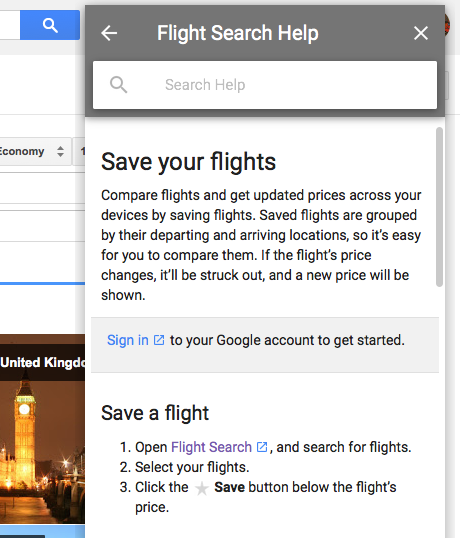The image depicts a cropped view of a website focusing on a pop-up window related to flight bookings. On the left side of the pop-up, there is a blue search bar adjacent to a blue search button. The background hints at a flight booking page, suggesting the user is in the process of booking a flight. Visible details include an 'Economy' button and references to the United Kingdom, accompanied by an image of Big Ben. 

The pop-up features a gray banner at the top labeled "Flight Search Help," with an arrow button and an X button for navigation and closing, respectively. Below this banner is a search bar labeled "Search Help." The main content of the pop-up is set against a white background with black text, providing detailed instructions. It informs the user that saved flights enable them to compare options and receive updated prices across devices, with price changes indicated by a strike-through and the updated price shown.

Highlighted in blue text, the pop-up prompts the user to "Sign in" via their Google account to begin saving flights. It explains the steps to save a flight: 1. Open the flight search via the provided link and search for flights. 2. Select the desired flights. 3. Click the star symbol (save button) below the flight’s price.